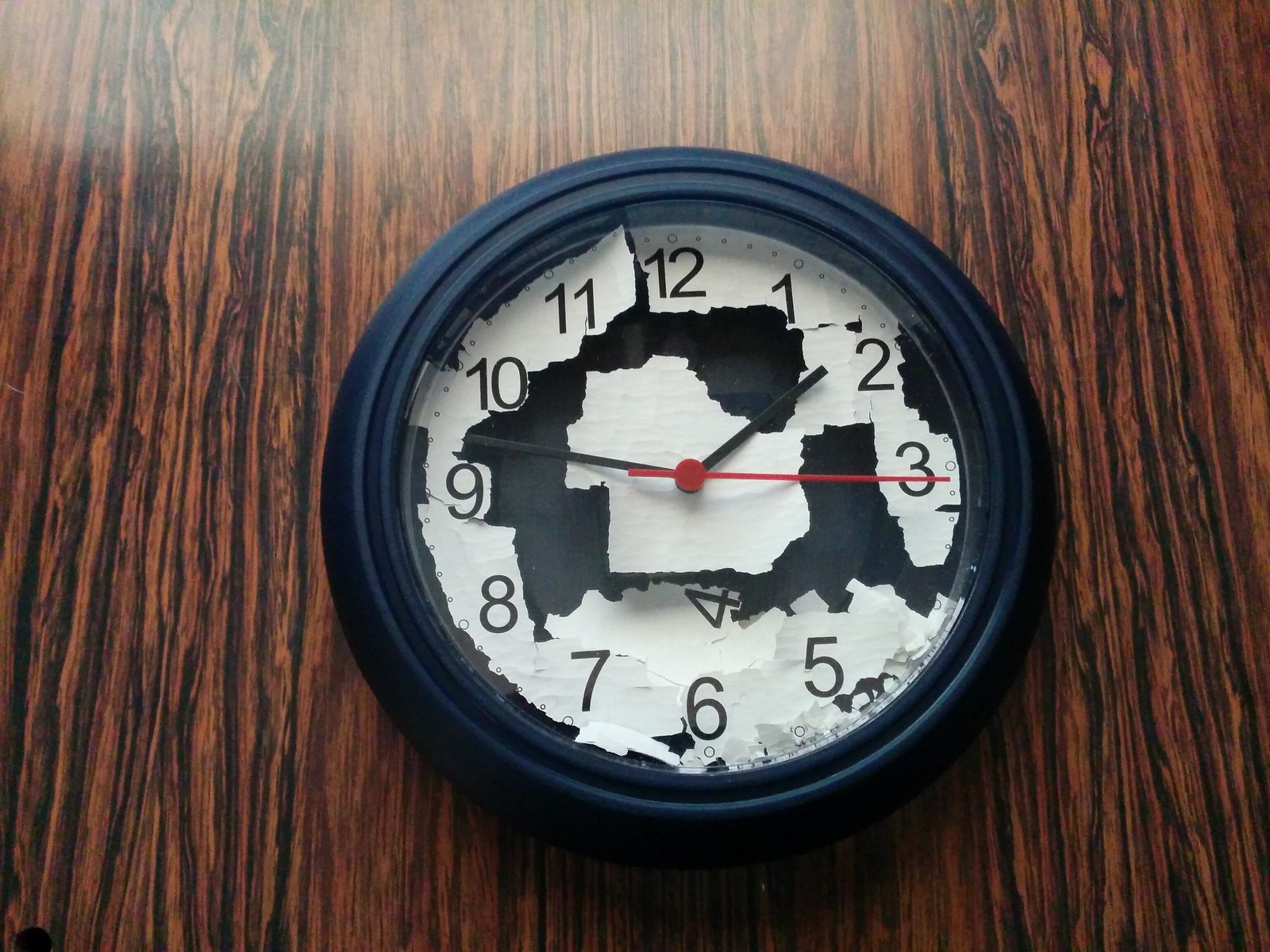This color photograph captures a round clock mounted on a piece of smooth wood paneling, positioned centrally within the frame. The clock has a black casing and a face that is notably deteriorating. The white clock face is peeling, especially noticeable at the top, with fragments accumulating at the bottom, creating a cluttered appearance around the six o'clock mark. The number four has detached from its original position and now rests directly over the six. The peeling paper has jagged edges, adding to the worn-out look of the clock. The hour and minute hands point around a quarter past either one or two, while the red second hand is positioned just below the three. The clock face also exhibits a mix of black, white, and blue hues, contrasting with the wood paneling behind it, which features shades of black and brown.